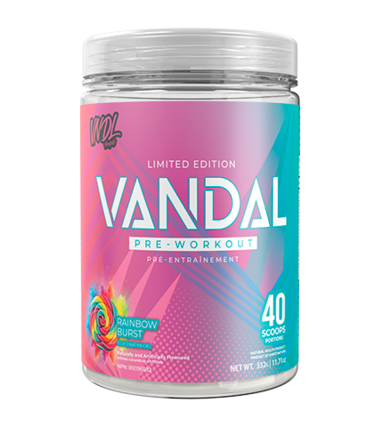The image depicts a round canister of a dietary supplement prominently placed against a white background. The canister features a silver cap and see-through glass body. The vibrant label displays a gradient transitioning from pink on the left side to turquoise blue on the right. The top left corner of the label bears the initials "VDL." Below this, in bold white text, it reads "Limited Edition Vandal," with "Vandal" outlined in blue. The label specifies the product as a "Pre-Workout, Pre-Entrenainment" supplement. At the bottom right, it notes "40 scoops," indicating the powdered form of the supplement. The left side boasts the flavor "Rainbow Burst," accompanied by an image of a multicolored lollipop. The canister appears to hold a net weight of approximately 300 grams.